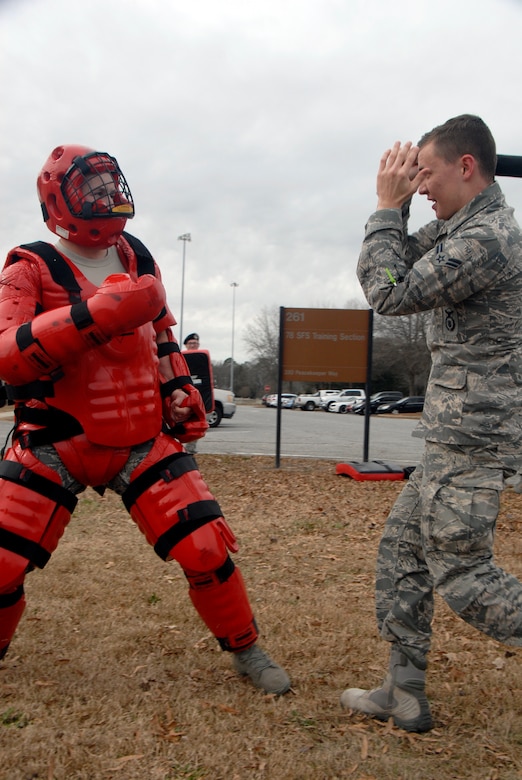In this detailed image, we see an outdoor scene centered on two military personnel engaging in physical training on a dry, brown grassy field. The focal point of the photograph is the sparring duo positioned right in the center of the frame. The man on the left is fully outfitted in a red padded bodysuit designed to absorb blows, complete with a protective helmet featuring a black cage-like face mask, boxing gloves, and various protective gear strapped to his body. The man on the right, dressed in a camouflage military uniform and wearing similar boots, stands ready with his hands guarding his face. This uniformed individual is identified as an airman first class, distinguished by the two chevrons on his Air Force stripe.

In the background, a parking lot lined with cars and an orange sign that reads "261-78-SFS Training Section" are visible, although the smaller text is hard to discern. Part of another person wearing a beret can also be seen behind the two main figures. The image is taken during a typical cloudy day, with the sky and clouds occupying the top of the frame, adding to the overall ambience of a routine training day. The color palette of the image includes hues of red, black, white, brown, green, orange, and gray.